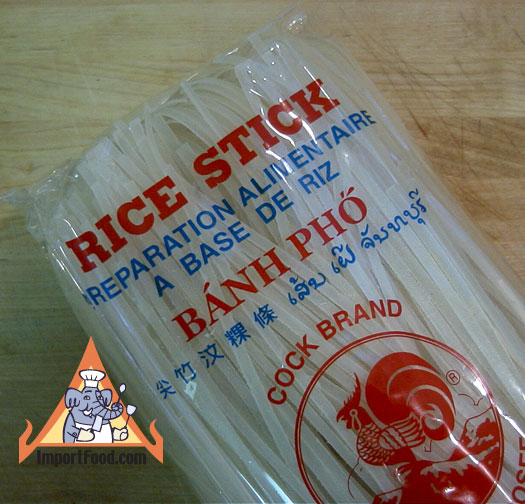In the indoor setting of this image, the background prominently features a light-colored cutting board with distinctive, darker grain patterns. Notably, the upper right section of the cutting board is marked with numerous slash marks that have turned gray due to discoloration. 

Positioned in the bottom left of the image is a triangular object, outlined in light orange with a very light yellow interior. This triangle showcases an anthropomorphic elephant, gray in color, standing in a humanoid pose facing the right. The elephant is attired in a white chef's hat and a white apron, holding a large cleaver in its left hand and a spatula in its right, both hands clad in white gloves. Beneath this whimsical depiction, the text "importfood.com" is printed in black.

Foregrounded in the image is a clear plastic bag containing what appears to be white, stringy rice sticks. The bag's labeling includes the term "Rice Stick" in red. It also displays "Banafo" in red surrounded by some blue Asian script alongside an additional segment of blue Asian script. Arching atop the bag in a curve is the word "Cockbrand," accompanied by an image of a rooster. The rooster, looking towards the bottom left, is red and enclosed in a red circle.